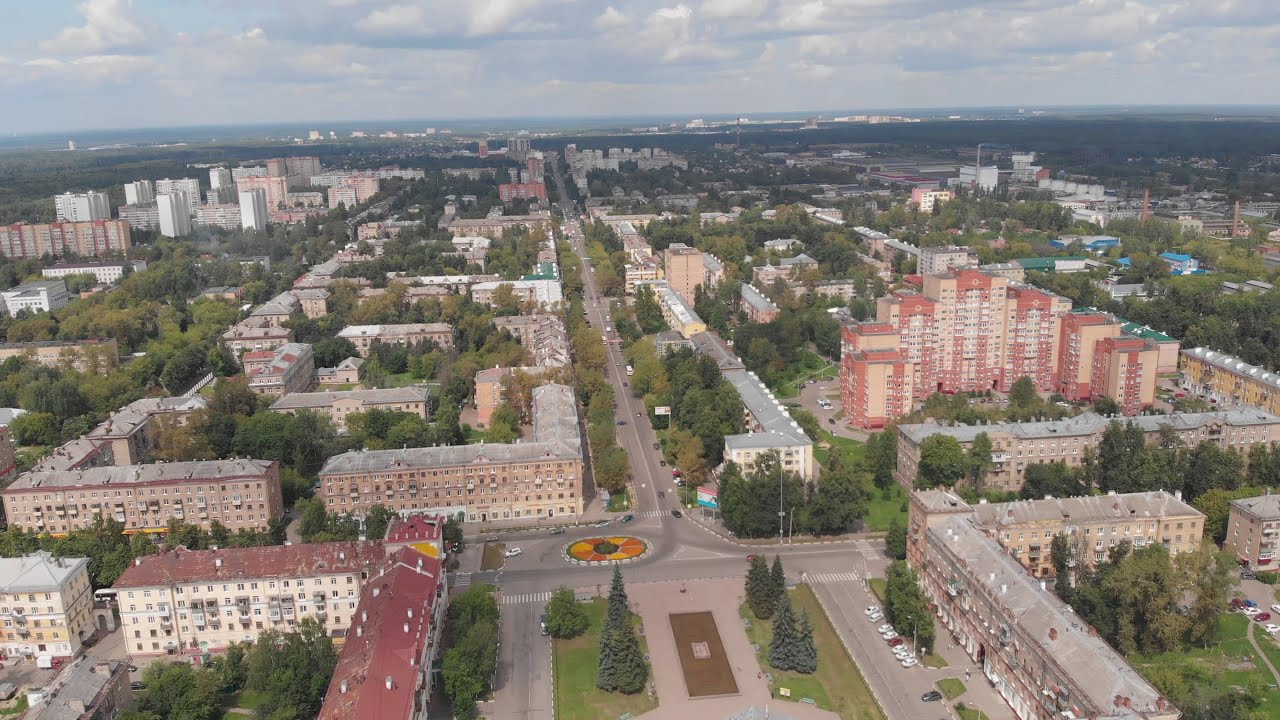The image captures an aerial view of a city under a cloudy, gray daytime sky. The top sixth of the picture features the city's skyline stretching from left to right, with distant buildings silhouetted against the horizon. The cloudy weather casts a dark shadow over the rear portion of the city. The central focus is a vertical two-lane street that divides the image, terminating in a T-section road. 

The city's landscape is composed of numerous multi-story rectangular brick buildings, many forming L-shapes at the corners of blocks. These buildings, predominantly apartment complexes with either red or gray roofs, border small green areas filled with trees and greenery, creating a picturesque urban environment. 

On the right side, there's a prominent taller structure, possibly a hotel or apartment building, characterized by its numerous windows. To the left, several additional apartment buildings are arranged in rows, each encircling a central park or garden area, enhancing the communal feel. Farther left in the upper portion of the image lies what appears to be the downtown area, distinguished by its taller buildings.

Trees line the main road, showcasing the city's blend of architecture and nature. The background features more buildings, possibly extending to a distant body of water, adding to the city's expansive, layered landscape.